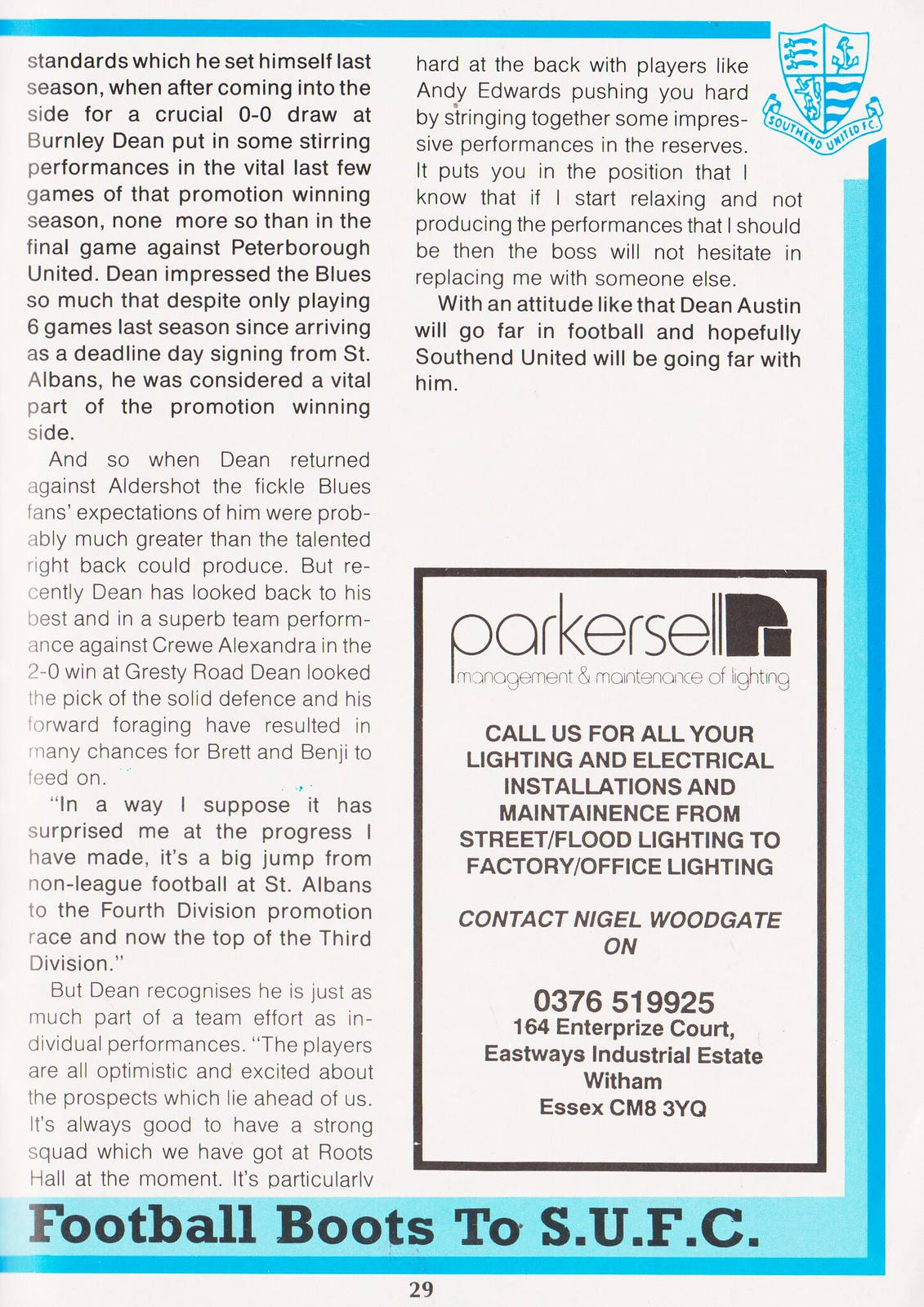This image shows a tall, rectangular page from a sports program, specifically page 29. The page is light gray with a bold blue border at the top and right edges. In the lower section, a lighter blue inner line runs along the bottom and right side. Within the light blue border at the bottom, bold black letters spell out "football boots to SUFC." 

The page is divided into two columns. The left column contains four paragraphs of small, black text, which include detailed descriptions of a player's performances and contributions to the team. A notable passage recounts how a player, Dean, impressed greatly in a final game against Peterborough United and was a crucial part of a promotion-winning season, despite limited appearances.

The right column starts with two paragraphs describing some more team-related information. Below these text blocks, in the bottom right corner, there is an advertisement. This ad is enclosed in a black rectangle, titled "Parker Cell," and contains several lines of text indicating various lighting and electrical installation services. Below the title, there's a section instructing readers to contact Nigel Woodgate, followed by a contact phone number and address.

An additional detail includes a dark blue emblem that looks like a coat of arms, situated in the upper right-hand corner, enhancing the page's formal and organized appearance.